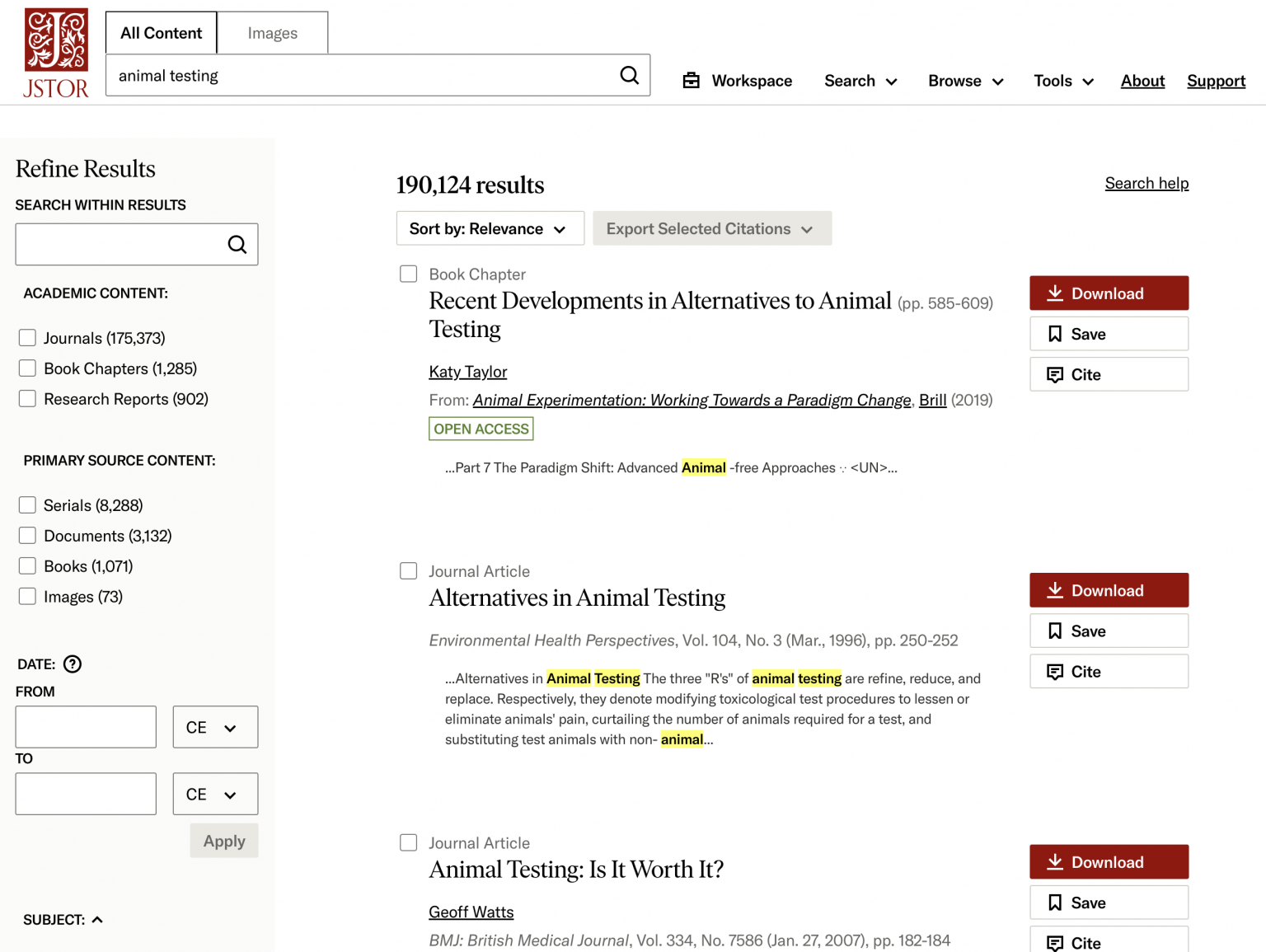**Detailed Caption:**
This image is a screenshot from the academic database JSTOR, showcasing its user interface. At the top left corner of the webpage, the JSTOR logo is prominently displayed; it features a red box with a stylized letter "J" entwined with vine-like designs. Directly to the right of the logo, a search bar is filled with the query "animal testing." The search bar has two tabs labeled "All Content" and "Images."

To the right of the search bar, a horizontal menu bar includes various navigational options: Workspace, Search, Browser, Tools, About (underlined), and Support (underlined). The main body of the webpage reveals the first three of 190,124 search results, sorted by relevance. The first result is a book chapter titled "Recent Developments in Alternatives to Animal Testing" by K.T. Taylor, marked with an "Open Access" tag. The second result is a journal article titled "Alternatives in Animal Testing," featuring highlighted instances of the search term "Animal Testing." The third result is a journal article "Animal Testing: Is It Worth It?" by Geoff Watts. Each article entry includes options on the right for downloading, saving, and citing, indicated by icons in red.

On the left side of the webpage, a floating sidebar titled "Refined Results" provides additional filtering options. This section includes a "Search Within Results" feature, with checkboxes for limiting results to journals, book chapters, and research reports under the "Academic Content" category. Another category, "Primary Source Content," lists options such as serials, documents, books, and images. There is also a date range filter and an "Apply" button for refining the search results even further.